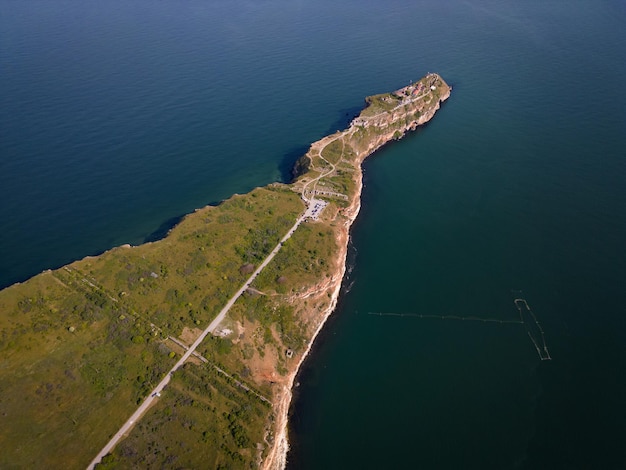This aerial photograph, likely taken from a drone or satellite, captures a small peninsula, possibly resembling the tip of Florida or an island in the Keys, surrounded by a vast expanse of dark blue water with hints of green near the shoreline. The peninsula stretches from the bottom left corner of the image and extends near the top right corner, stopping slightly over halfway through the frame. The land is densely green with patches of grass and trees, interspersed with some shrubbery, and features a prominent road running through the middle, leading to the tip of the peninsula. In the center of the landmass, there’s a distinguishable parking lot with a few visible cars. On the right side of the image, a faint dock or pier extends out into the water, inviting speculation about its exact nature. The scene is bathed in subdued daylight, suggesting it might be later in the day.